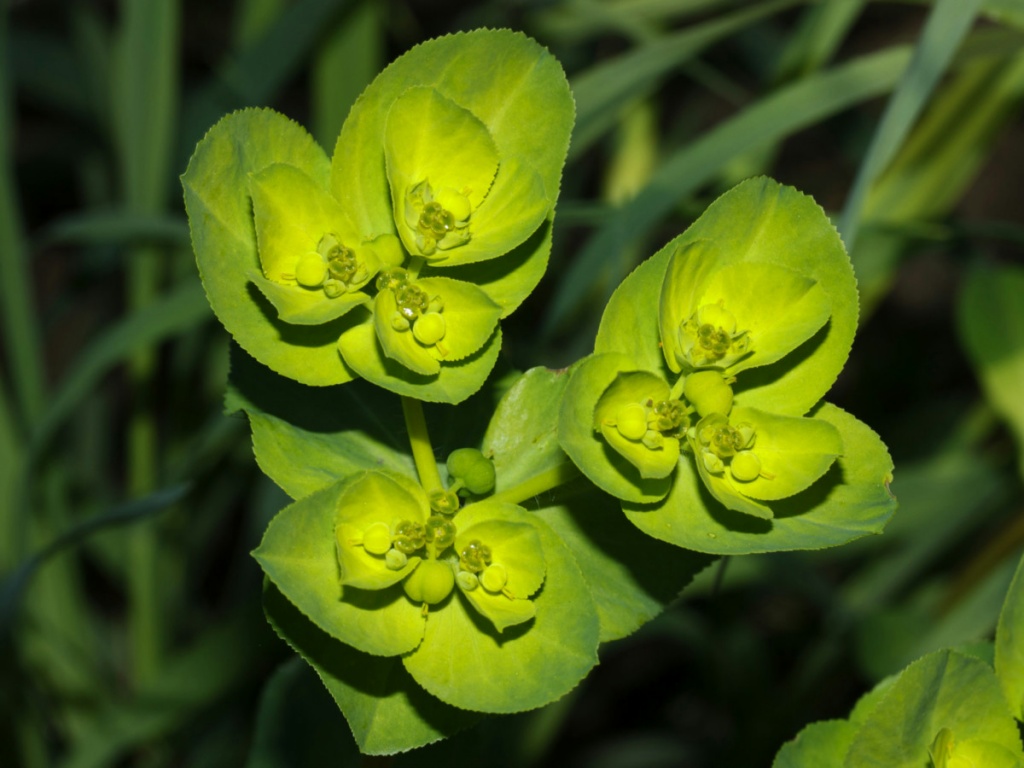This image captures a detailed close-up of a lush green plant in landscape orientation. The main focus is on three central plant heads, each emerging from their own small stalk and surrounded by a myriad of leaves. The plant heads are more luminous compared to the darker, nearly black voids in the background, providing a striking contrast. Each plant head boasts layers of leaves - some larger, some smaller - and among these leaves are small, dark buds, with about three to four buds per plant head. These buds resemble tiny, miniature apples in shape and are covered with a fuzzy texture. The color palette varies from dark green to a light yellowish-green, adding depth and richness to the image. The background is slightly blurred, revealing slender, long strands of grass and additional leaves, all contributing to the overall green theme of the photograph.